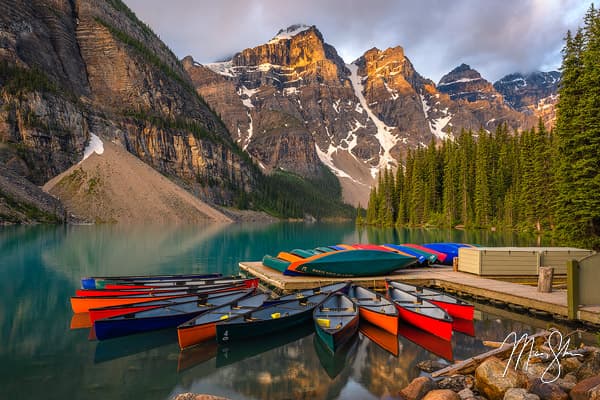This photograph captures a serene mountain lake scene, dominated by a wooden dock situated almost at the center of the image. The dock is adorned with an array of colorful kayaks and canoes, boasting hues of red, orange, dark green, and dark blue. Some vessels rest atop the dock while others gently float in the calm, highly reflective blue water. The scenic beauty extends to the background, where imposing mountains with patches of lingering snow and exposed rocky crags rise majestically. The mountainsides are densely forested with clusters of tall pine and conical evergreen trees. The sky overhead is a tapestry of dark gray clouds interspersed with glimpses of blue, allowing sunlight to filter through and bathe the landscape in a soft glow. A barely discernible photographer's watermark, written in script, is located in the bottom right corner of the image. This picturesque scene harmoniously blends natural elements, showcasing the tranquil essence of a mountain lake amidst thriving wilderness.